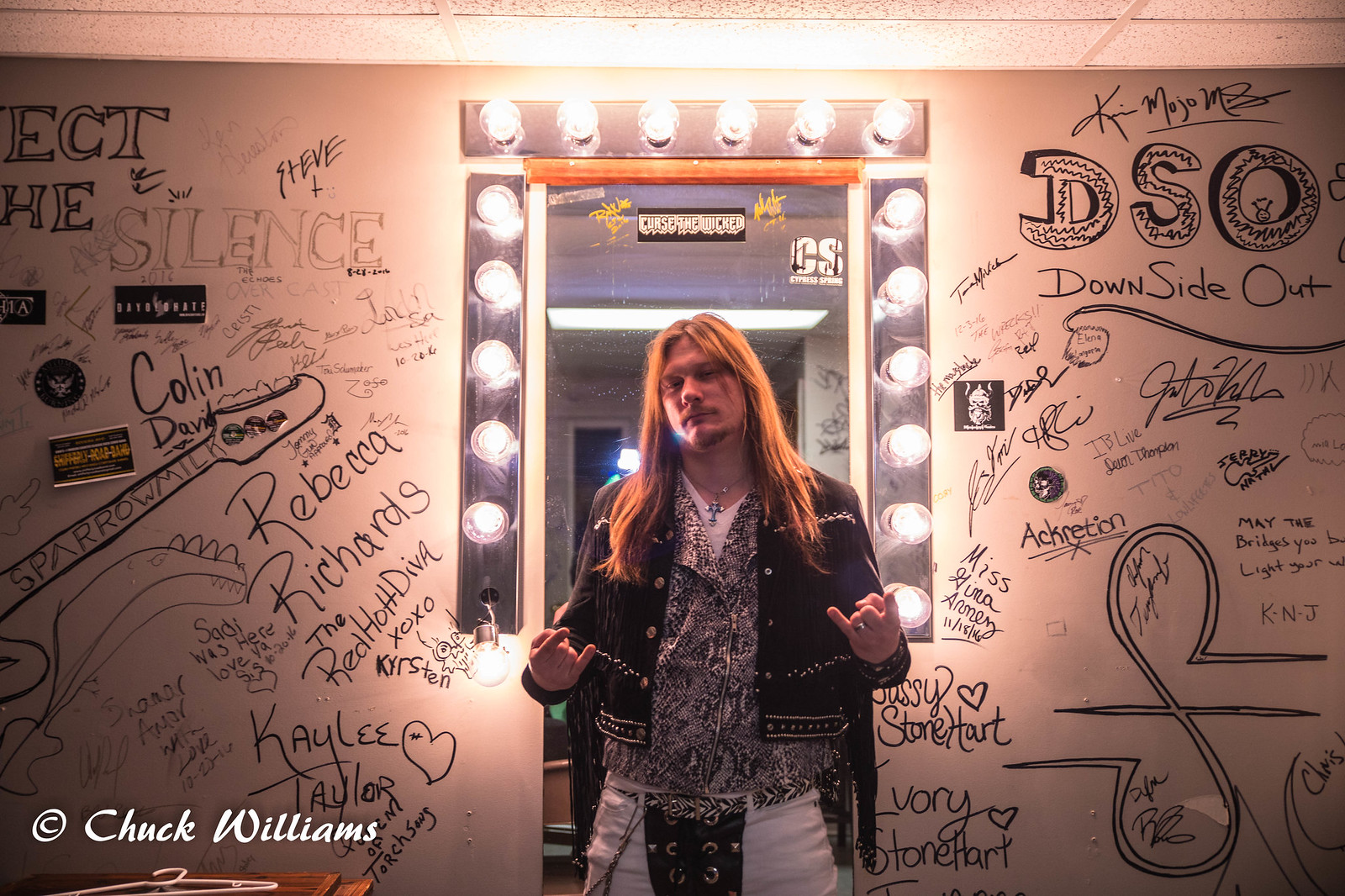In this vibrant dressing room scene, a rock star with long, dirty blonde hair and a goatee takes center stage. His eyes are squinted, and his expression is one of confident intensity. He wears a silver cross necklace, layered outfits including a black short jacket over a snake skin or zebra print vest, and a white V-neck T-shirt. His white pants feature a tied crotch piece and a chain by his pocket. The man holds up the iconic "devil horns" hand gesture. Behind him, a large mirror with surrounding light bulbs illuminates the space. The white wall behind and around the mirror is densely covered with signatures, graffiti, and drawings, including prominent names like Downside Out, Rebecca Richards, and Kaylee Taylor, who have added their marks in various colors. Some graffiti features yellow designs, adding to the room's colorful chaos. In the lower left corner, the text reads "Chuck Williams," suggesting the room's ownership or the photographer's credit. The whole ambiance exudes the edgy, electric vibe of the rock and roll lifestyle.